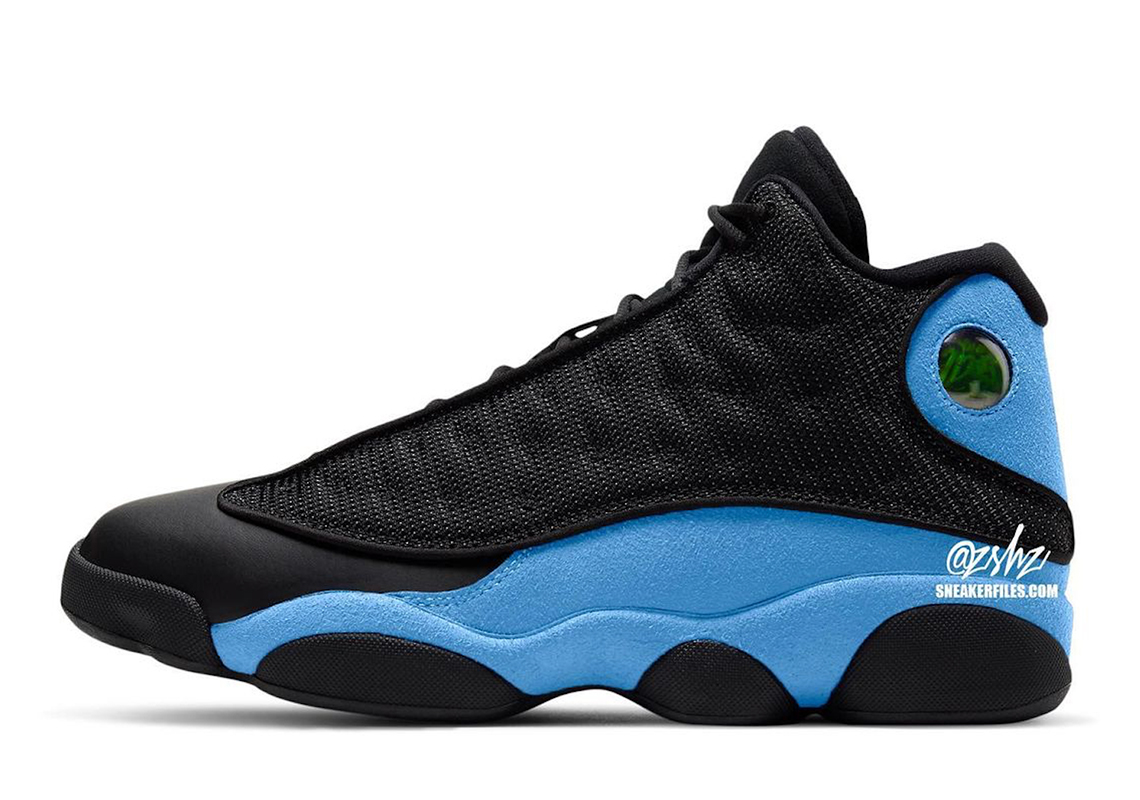This detailed image features a close-up, profile shot of a high-top sneaker against a white background, casting a shadow underneath it. The sneaker exhibits a striking design with a distinctive color split: the toe, tongue, and upper sections around the laces are black, while the sides and portions of the back of the shoe are a light blue. Notably, a blue design with a clear plastic circle adorns the ankle area, and a blue pattern with half-circles encircles the shoe's footbed near the sole. The laces are tucked in, obscuring their length. On the right side of the sneaker, near the bottom, is a white, blocky font inscription that reads "sneakerfiles.com," along with an at symbol and some letters, likely "ZSHZ." This combination of colors and details contribute to the sneaker’s unique and modern aesthetic.